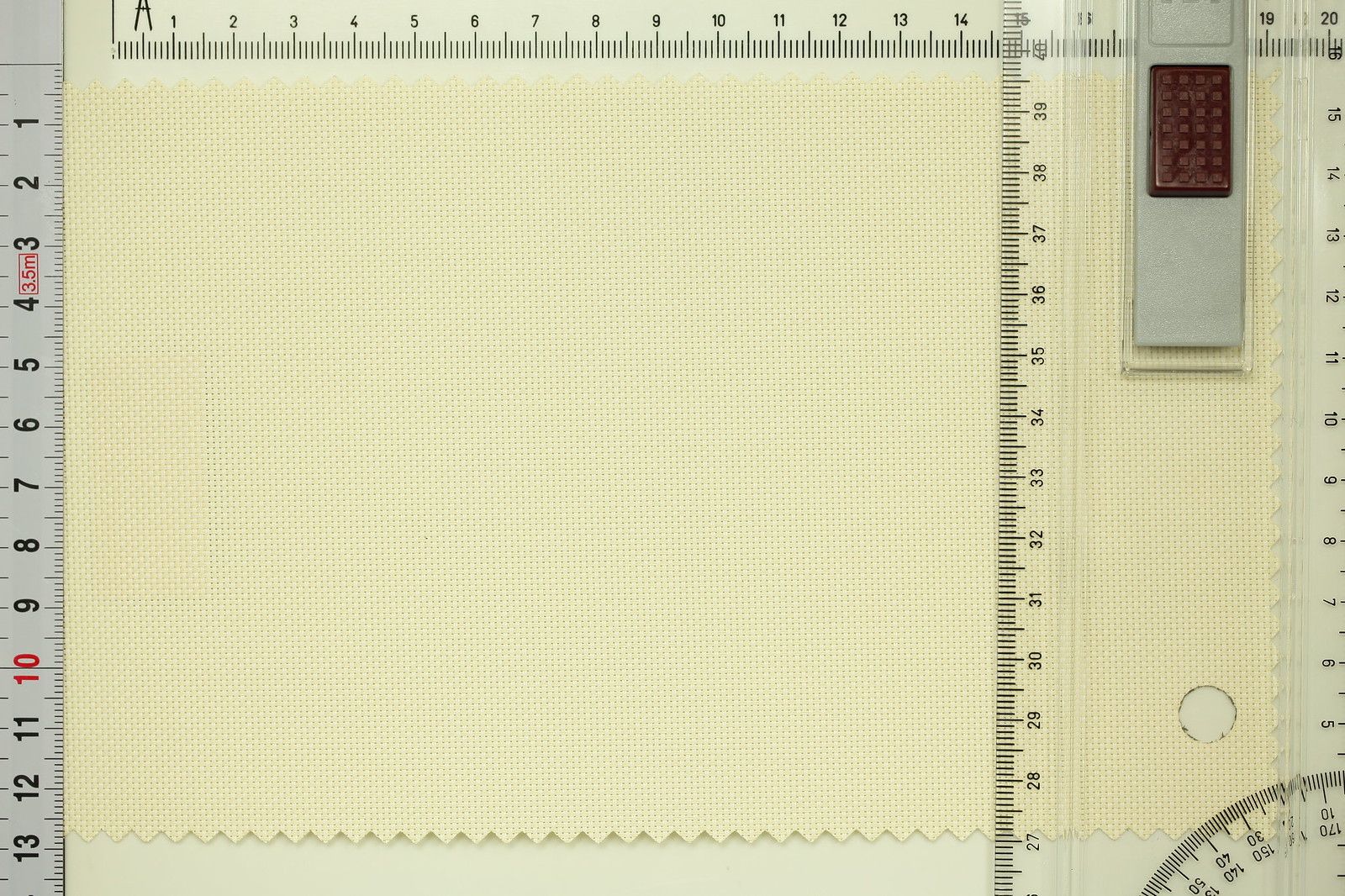This photograph features a detailed, organized workspace, possibly a drafter's table or an area dedicated to fabric cutting or crafting. The main focal point is a piece of ivory fabric with a woven texture and zigzag cut edges, positioned on a clean white tabletop. Surrounding this fabric is an array of measuring tools; a roller on the left provides incremental measurements from 1 inch to 13 inches, and another roller on the right measures up to 20 inches in similar increments. 

A prominent clear plastic measuring tape runs along the right side of the fabric, and there is another rounded measuring guide in the lower right corner, likely for adjusting angled cuts. Additionally, there's a ruler at the top edge of the workspace running horizontally from left to right, and another along the bottom edge. 

In the upper right corner, a solid gray rectangle is visible, topped with a smaller dark brown rectangle, resembling a mini chocolate bar, possibly a small tool or part of the workspace's equipment. This comprehensive setup suggests an environment designed for precision, whether for drafting, fabric cutting, or architectural work.